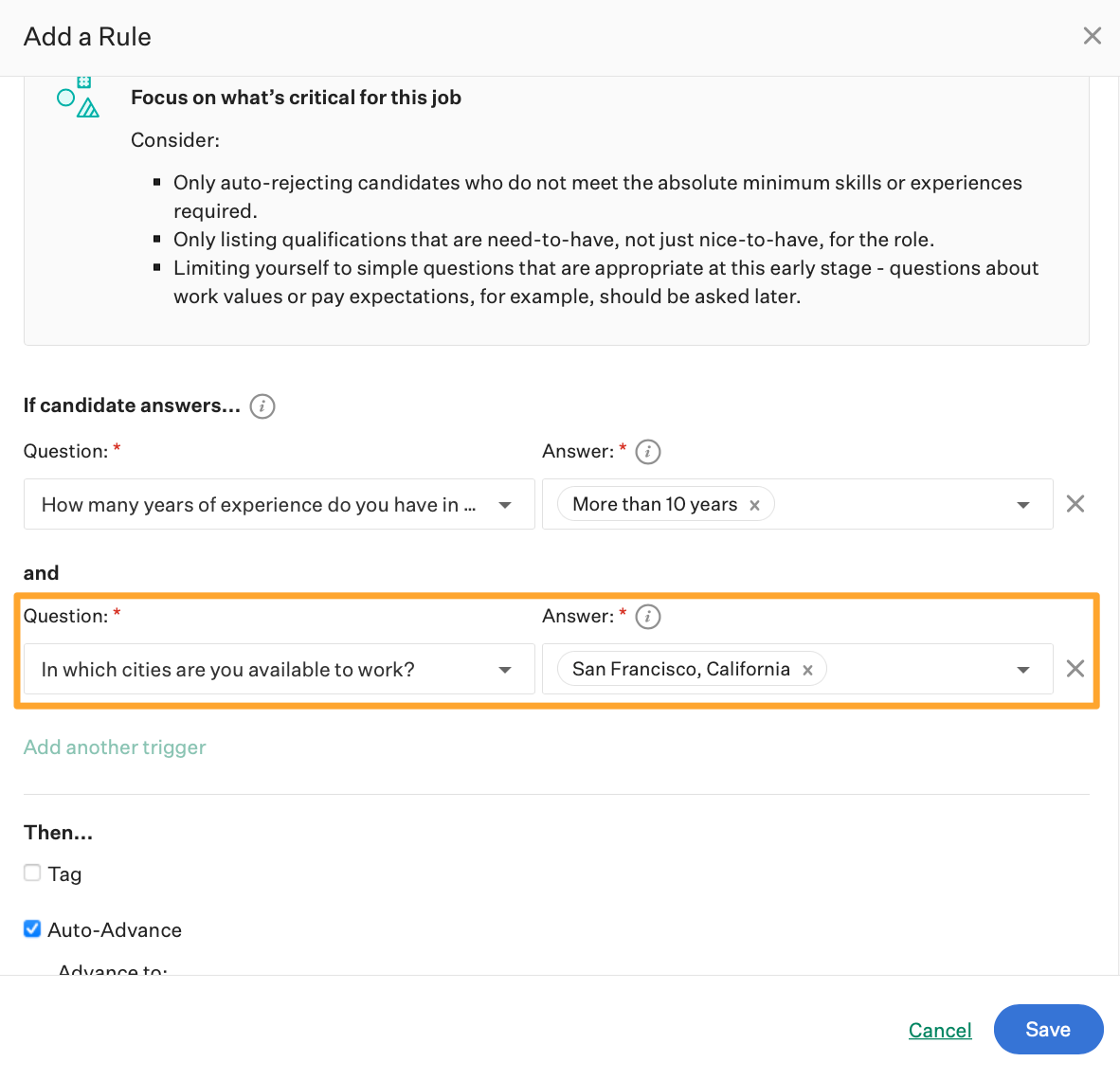**Caption:**

At the top of the webpage, there's a narrow, almost off-white bar featuring the text "Add a rule" on the top-left corner, countered by an 'X' on the top-right. Below this, a slightly darker gray box spans across with an array of icons on the far left—triangle, square, circles, triangle—followed by black text stating "Focus on what's critical for this job." Directly underneath, in unbolded font, it reads "Consider:" introducing a set of bullet points:

1. Only auto-rejecting candidates who do not meet the absolute minimum skills or experiences required.
2. Only listing qualifications that are 'need to have,' not just 'nice to have' for the role.
3. Limiting yourself to simple questions that are appropriate at this early stage; questions about work values or pay expectations, for example, should be asked later.

Further down, there are several drop-down boxes. A bolded heading reads "If the candidate answers," followed by "Question" and "Answer" each paired with their respective drop-down boxes. Under the "Question" section, it asks "How many years of experience do you have in," accompanied by a drop-down box for field specification. Under "Answer," there's a small bubble indicating "More than 10 years," which can be edited or removed as needed. Below, another bolded heading with the same question-answer format is present, this time marked by an orange box around the second Q&A field.